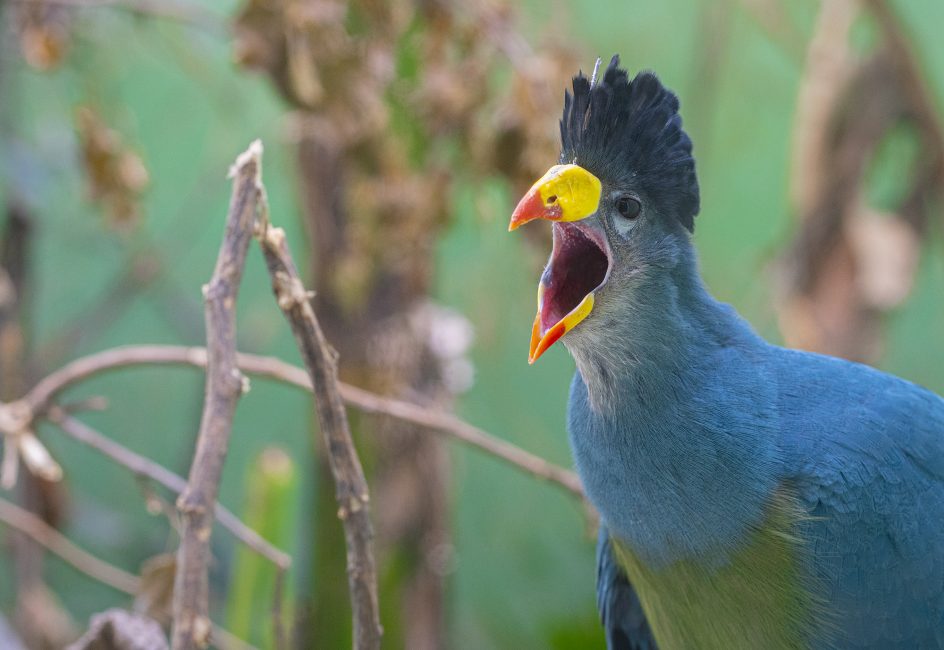This photograph captures a vibrant outdoor scene featuring a great blue turaco prominently positioned in the bottom right corner. The bird, adorned mostly in striking blue feathers with a green-feathered chest and a tuft of dark blue feathers crowning its head, is depicted mid-screech with its mouth wide open, revealing a pinkish interior. Its expressive face is framed by a ring of whiter feathers around the eyes and below the neck. The turaco's distinctive beak, which is predominantly yellow with a red tip, and its stark black eyes add to its vivid appearance. The bird's posture allows a partial view of its wings; the left wing slightly lifted, showing its underside, while the right wing remains folded. Surrounding the turaco are upright twigs, with additional branches discernible to the left side of the image. The background fades into a blur of trees, trunks of gray and light brown, and patches of green grass and leaves, enhancing the natural, serene ambiance of the photograph.